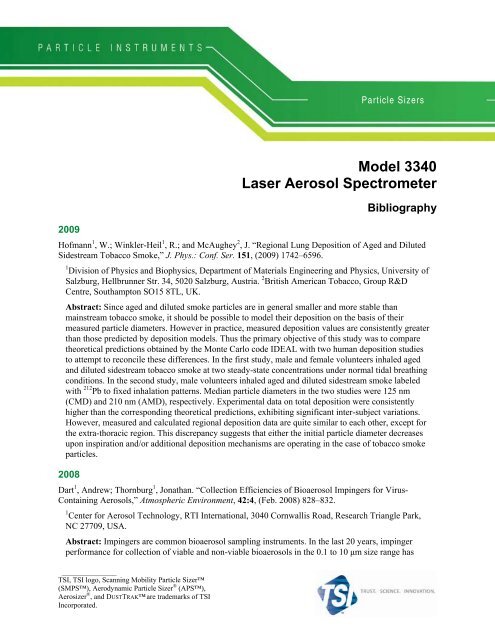This photograph portrays a detailed page likely from a catalog or technical document. At the top, a distinct green banner with white text reads "Particle Instruments Particle Sizers." The banner is straight, dips down diagonally in the center, and straightens out again. Below it lies another thin green bar and a white strip mirroring this stepped pattern. Prominent black text beneath these bars announces the "Model 3340 Laser Aerosol Spectrometer," with "Bibliography" following.

The page is divided into two sections for the years 2009 and 2008, each section beginning with the respective year in green text. Under these headings, there is a list of what seem to be bibliographic entries or references, totaling around 20 to 30 lines of small black text. Notably, each section appears to include detailed names and potentially the titles of works related to the device. Additionally, the lower right corner of the page features a blue logo with the letters "TSI" set within a diamond-like shape. At the bottom, a small, blurry section seems to mention "trademark" information. The overall presentation conveys a formal and structured documentation format for a specialized instrument.